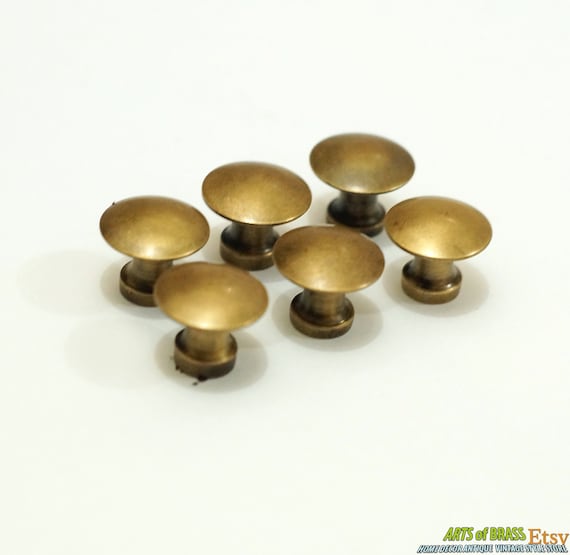The image features six shiny brass doorknobs or drawer pulls, each with a round, slightly flat top, and a smaller round base beneath. They are arranged upright in two neat rows of three on a plain white background, resembling a miniature egg carton. These doorknobs are golden in color and appear to be half of a traditional doorknob, showcasing the curved handle part. The bottom right corner of the image displays the text "Arts of Brass" in green, with "Home Decor Antique Vintage Style Store" written in white lettering with blue outlines below it. There's also an "Etsy" logo in orange nearby.